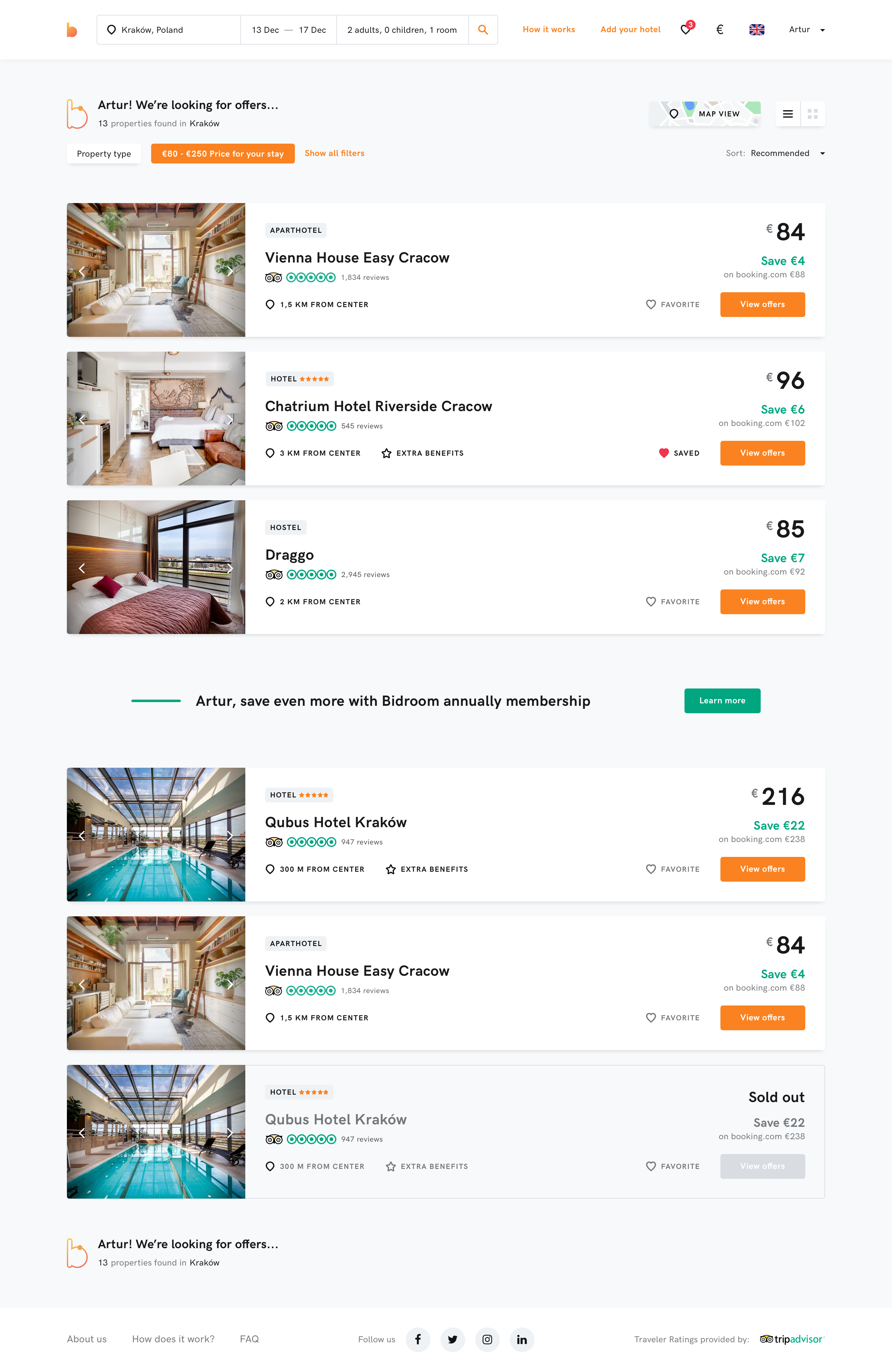The image depicts a user interface on a hotel booking website, showcasing various accommodation options in Krakow. The site features a white or light grey background with orange buttons for easy navigation. Displayed prominently at the top is a logged-in user profile named "Artur," indicating that the user is currently signed in and browsing hotel offers. The listings include detailed interior shots and span several price ranges and hotel names:

1. Vienna House Easy Krakow, priced at €84 per night.
2. Chatrium Hotel Riverside Krakow, listed at €96 per night.
3. Drago Hotel, with a rate of €85 per night.
4. Multiple listings for Cubis Hotel, with one highlighted option, Cubis Hotel, priced at €216 per night, showcasing a huge Olympic-sized swimming pool.

The design of the website is clean and user-friendly, allowing easy access to various hotel options in Krakow.